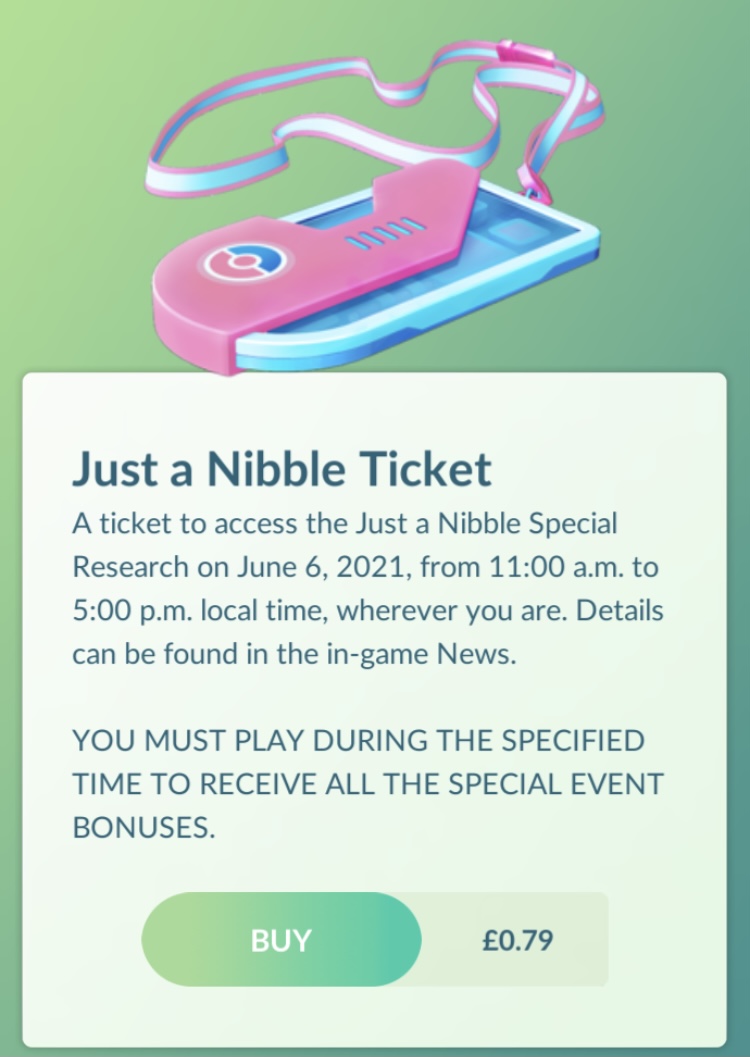This image is a screenshot of a website page featuring a promotional offer for an online game event. The background of the screenshot displays a harmonious gradient, transitioning from a lighter green on the left to a darker green on the right. At the top center of the image, there is a small, pink-colored object, which appears to be encased in a cover and attached to a lanyard, suggesting it is an in-game item.

Below this object, there is a rectangular, light greenish-yellow box containing text. The text reads "Just a Nibble Ticket" and describes it as a ticket granting access to the "Just a Nibble Special Research" event, scheduled for June 6, 2021, from 11 a.m. to 5 p.m. local time, regardless of the user's location. For additional details, players are directed to check the in-game news. 

Emphasized beneath the event description is an all-uppercase warning: "YOU MUST PLAY DURING THE SPECIFIED TIME TO RECEIVE ALL THE SPECIAL EVENT BONUSES."

A prominent button labeled 'Buy' is positioned below the text, indicating the ticket's price at £0.79. The central portion of the image, housing all the informative text and button, is predominantly a yellowish-green color with a slight tilt towards yellow, and it occupies approximately two-thirds of the overall picture.

The image's font is clear and appealing, suitable for conveying game-related information. Overall, this promotional screenshot effectively highlights the special event and encourages players to purchase the ticket while emphasizing the importance of participating within the specified timeframe.